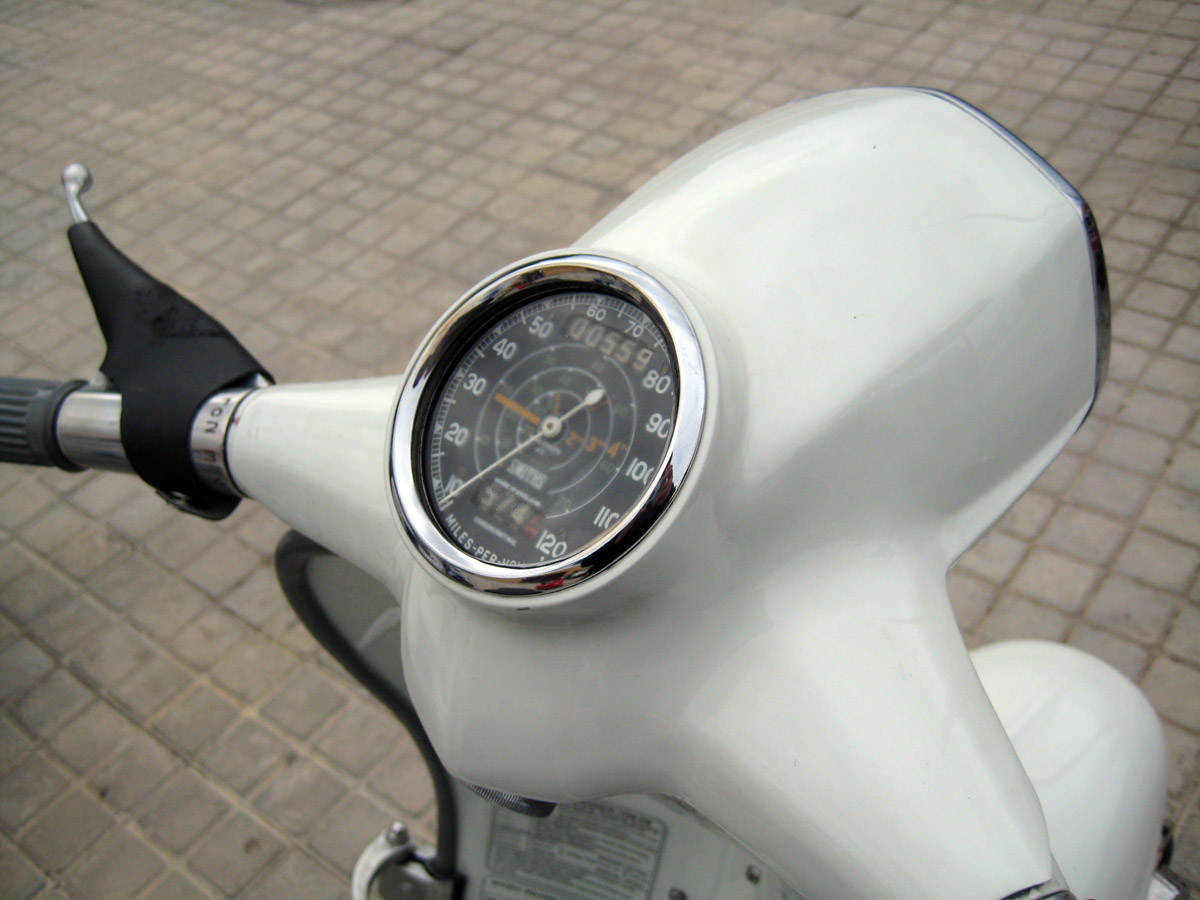The image features a sleek, white European scooter parked on a quaint brick-paved street. The handlebars, entirely encased in pristine white plastic casing, conceal all wiring underneath, giving the scooter a clean and streamlined appearance. Accentuating the center of the handlebars is a prominent speedometer, bordered by a stainless steel ring. The face of the speedometer is black, adorned with white numerals in increments ranging from 10 to 120. A white needle serves as the indicator for speed. While the picture is taken from a side and overhead angle, making the bottom numbers somewhat difficult to discern, both digital readouts at the top and bottom of the speedometer can be seen. The scooter's elegant design and meticulous casing evoke the stylish and practical aesthetic synonymous with urban European transport.